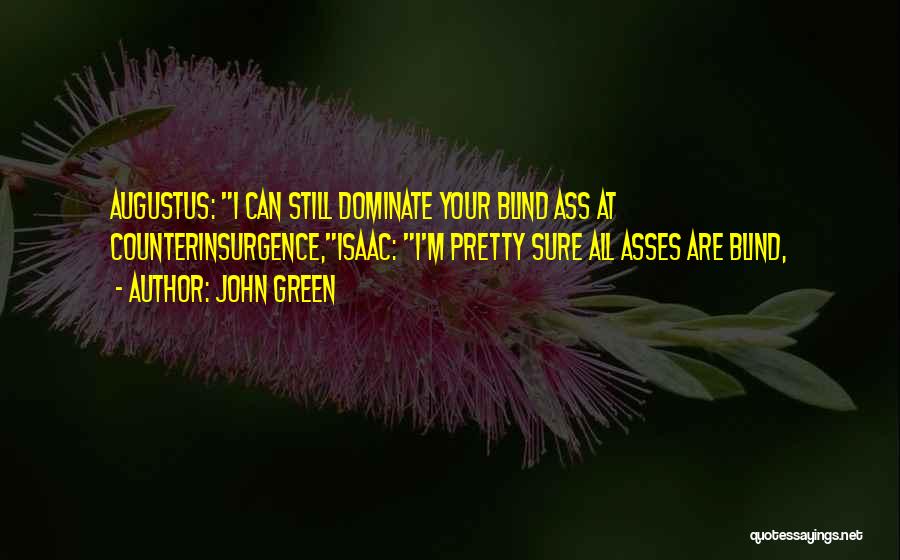The image features a quote in bright yellow text set against a very dark, black background. In the center of the image, the quote reads, "Augustus, I can still dominate your blind ass at counterinsurgents. Isaac, I'm pretty sure all S's are blind." The author is identified as John Green. The background is a very dim, darkened image of a pink flower with small green leaves, almost thorny in appearance, resembling a cactus flower. The flower is slightly visible, adding a subtle visual element to the dark theme. In the bottom right corner, "quotessayings.net" is written in white text. The overall image has an ominous feel, with the yellow text standing out as the only bright element.